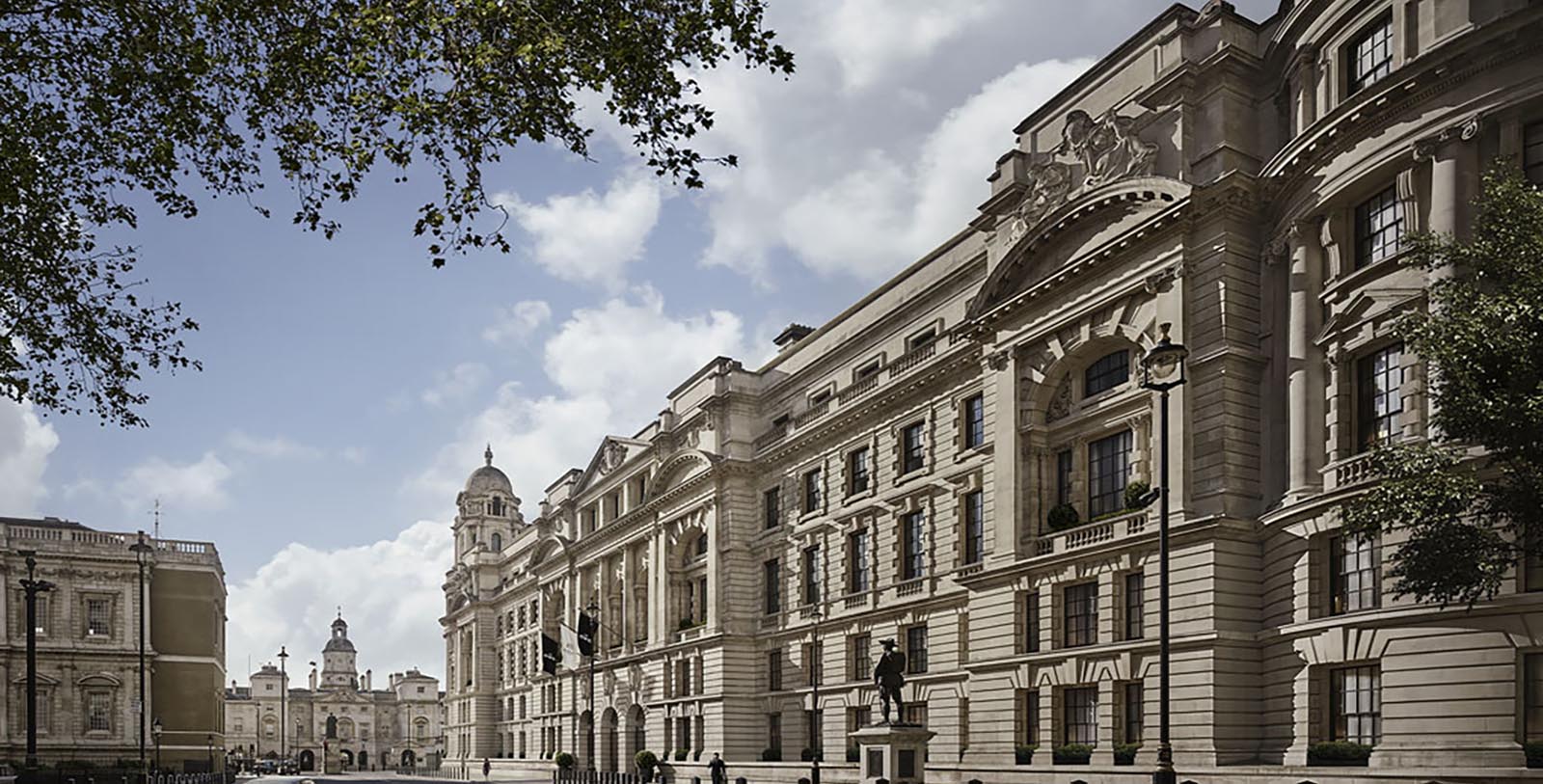This image depicts a grand, five-story tan stone building featuring British-style architecture, with numerous windows, balconies, and ornate carvings above arched entrances. The facade is complemented by large columns and three prominent arches at the center, marking the main entrance, which is accentuated by two dark flags. In front of this elaborate structure stands a small, black statue, possibly of a man, although the details are unclear. The scene is enriched by a domed tower in the background, suggesting a church-like building, and additional similar architectural styles are visible in the distance. On the far right, the photograph captures the vibrant green leaves of a tree, and more foliage appears in the top left corner. The sky above is a cloudy blue, enhancing the stately atmosphere of the setting.